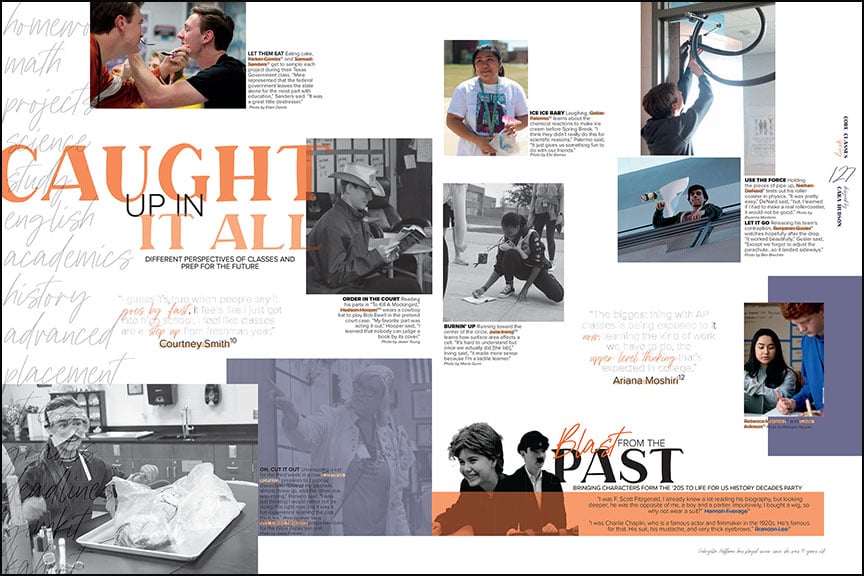The image in landscape mode is a detailed and vibrant print ad, featuring a collection of inset pictures presented in both black and white and color. Dominating the left side, an orange text reads, "Caught up in it all," with a black subtitle underneath stating, "Different perspectives of classes and prep for the future." 

The collage of images includes:
- A black and white photo of a young boy in a cowboy hat engrossed in reading a book.
- A black and white image of a girl kneeling on an outdoor sidewalk, seemingly absorbed in writing in a white book.
- A color photograph capturing a person on a balcony, mid-action as they toss an object off the side.
- A color image of a teenage boy and girl collaborating on writing something together.

This ad is visually stimulating with its white background and each photo is accompanied by captions in black text, highlighting one or two crucial keywords in orange, enhancing the thematic elements and drawing the viewer’s attention to the diversity of activities and perspectives showcased.